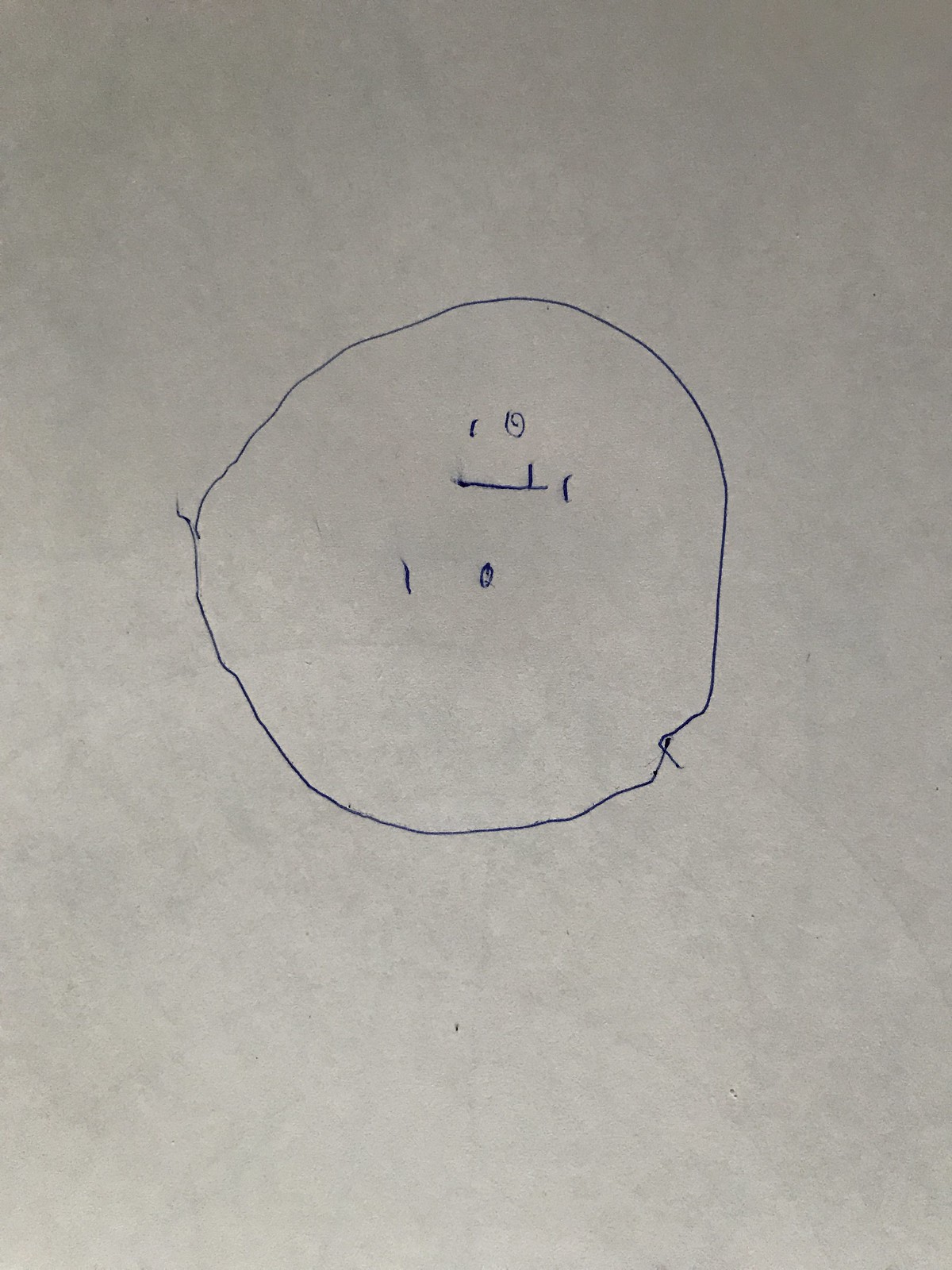A piece of grayish construction paper is displayed with visible fibers embedded within its surface, indicating it's not particularly clean. Near the center of the paper, a child-like doodle is discernible, made with a blue ballpoint pen. Though the drawing appears as a series of random dots and lines in its current orientation, a 90-degree rotation reveals it to be a simplistic yet charming depiction of a face, complete with two eyebrows, two eyes, a nose, and a mouth. The amateurish nature of the artwork suggests it was likely created by a young child, possibly a kindergarten student. The photograph captures this innocent creation, albeit oriented incorrectly.